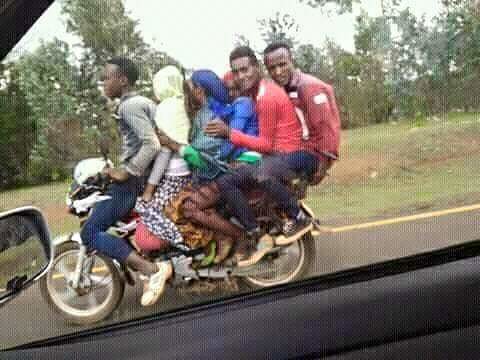The image captures a remarkable and somewhat precarious scene of six adults, a mix of three men and three women, straddling a single motorcycle as it drives along a paved road. The motorcycle is closely aligned with the yellow line marking the edge of the road, surrounded by a field of grass and a line of green trees. Above, a cloudy sky hints at an overcast day. This shot, angled slightly from the passenger side window of a gray car, includes part of the car's interior and its side mirror in the frame. The riders, all with dark skin and dressed in various colors including blue, red, and gray, cling to one another. The man in the front, steering the bike, wears blue pants and a gray top, while the others look either ahead or to the side, with one person smiling amidst the unlikely scene.